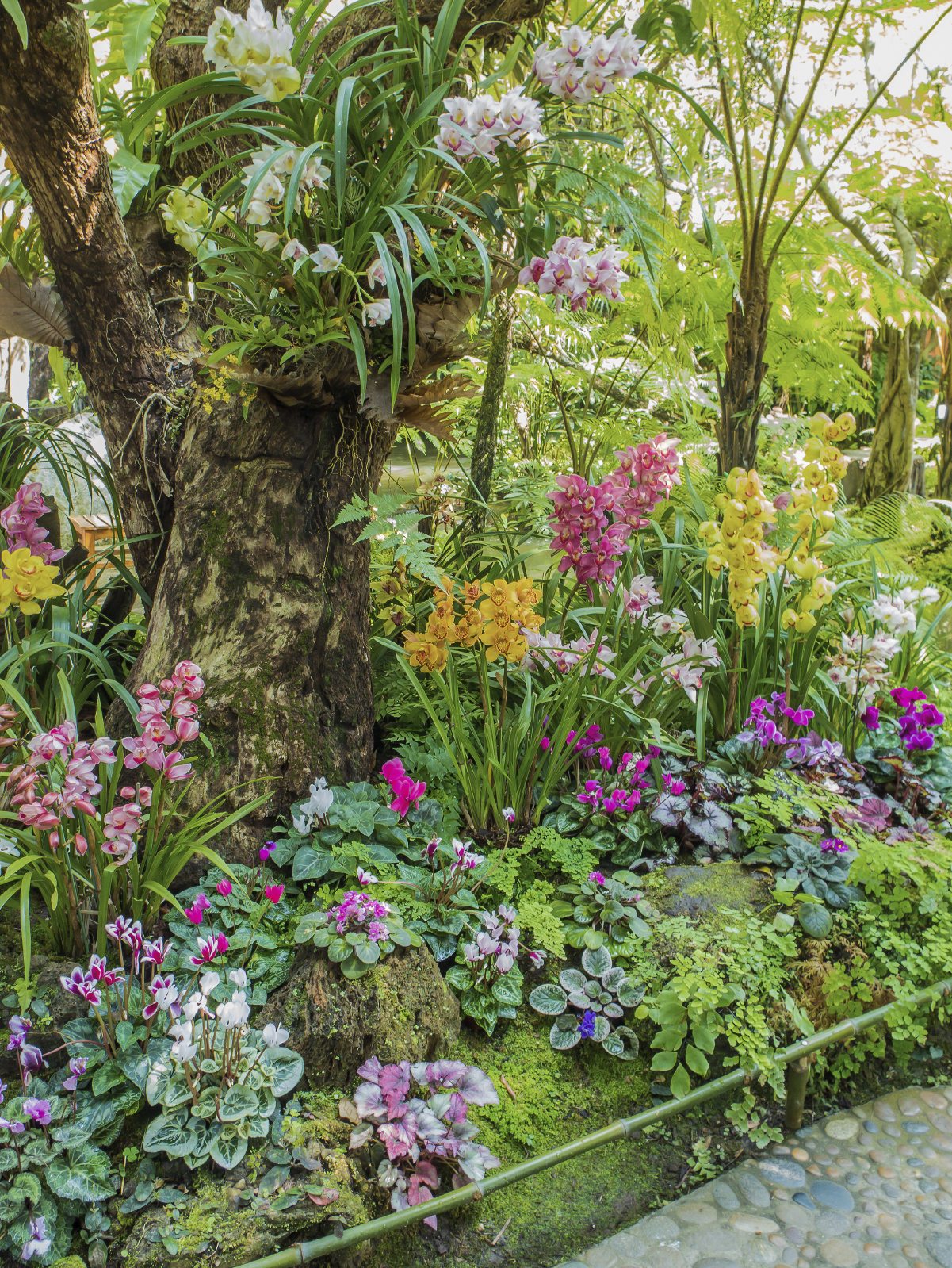This image captures a vibrant and meticulously curated tropical garden, likely part of a zoo exhibit or a nature reserve within a park. It showcases a lush area full of diverse flora, with a dominant tree on the left adorned with vining and flowering plants. The garden is replete with colorful flowers in a spectrum of shades, including yellow, pink, purple, white, and even lilacs and blue hues. The foliage is a rich tapestry of greens, from lighter algae-like growths to darker variegated leaves. The scene is completed by a cobblestone walkway visible in the bottom right, inviting visitors to leisurely stroll and immerse themselves in the natural beauty of this picturesque setting.